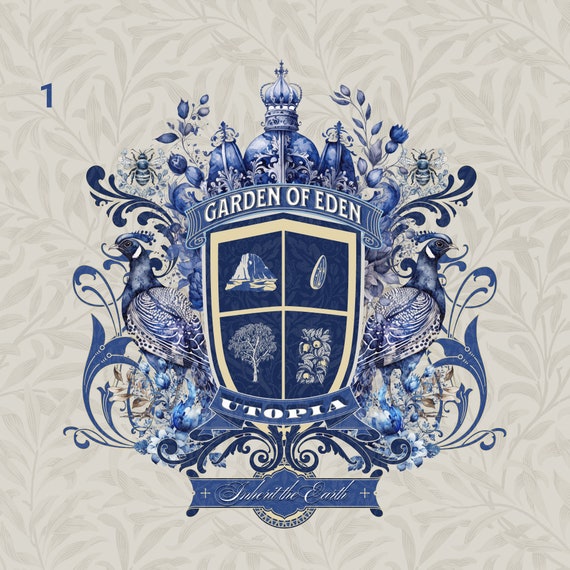The image depicts a detailed, printed emblem against a gray background with graphic leaf patterns. Central to the composition is a blue and white shield prominently featuring four distinct panels: one with a tree, another with a mountain, a third with a plant bearing fruit, and a circular object in the last. Above the shield, the words "Garden of Eden" are inscribed, while "Utopia" is written below. Crowned at the top, the shield is flanked by two birds—resembling partridges or pheasants—facing each other in profile. Adorning the edges of the emblem are intricate flowers and curlicues, enhancing the ornamental quality of the piece. Additionally, two bees are positioned near the top of the emblem. Beneath the shield, a blue banner bears the inscription "Inherit the Earth" in white script, though somewhat distorted and challenging to read clearly. The overall image is crisp, utilizing natural light, and its primary color scheme is blue and white.